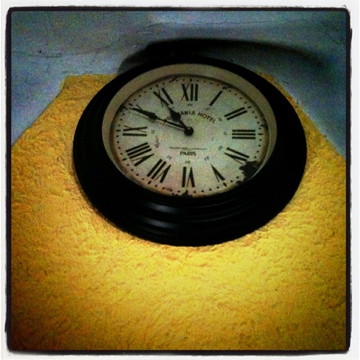The photograph features an analog clock embedded in a yellowish foam substance, likely house insulation. The clock's surface is reminiscent of an upside-down bowl, curving outward from its base. Above the clock, there is a curved white surface, possibly made of metal or concrete. The clock face displays Roman numerals from I to XII, encircling the dial. Two black hands with pointed ends, resembling the spades from a deck of cards, indicate the time is approximately 10:50.